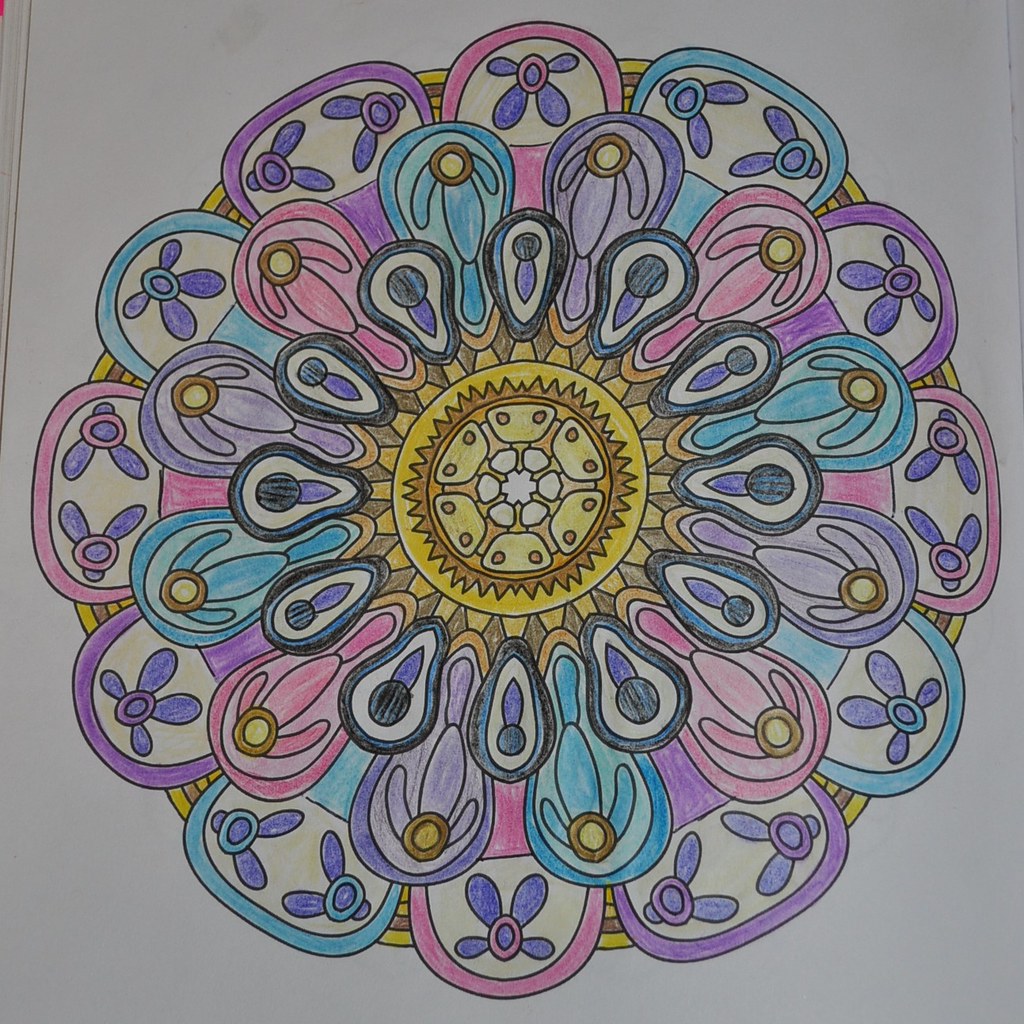The image depicts a vividly colored, mandala-like design that resembles a flower, rendered with colored pencils. At the heart of the mandala is a sun-like central shape, colored in bronzish-yellow, featuring a smaller white flower within. Radiating outward from this central point are three distinct layers of petal-like shapes arranged in circular rows, giving the overall design a sense of movement and depth.

The innermost layer consists of narrow, dark blue and white petals with a purple center. The middle layer showcases alternating petals in shades of pink, blue, and purple. The outermost layer continues this alternating color scheme of pink, blue, and purple petals. Each petal also has a detailed design of its own, some resembling three- or four-pronged flowers.

Surrounding the petals and providing a border to the design is a yellow outline against a white background, which is indicative of sketch paper. The color palette includes vibrant purples, blues, pinks, yellows, browns, and blacks, contributing to a psychedelic and intricate appearance.